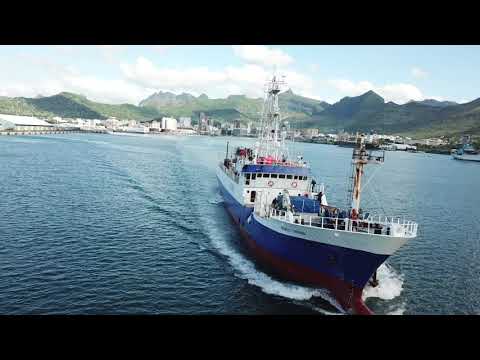An aerial or drone shot captures a bustling commercial boat at the center of a picturesque bay, heading towards the viewer at a slight angle. The boat features a distinctive white, blue, and red striped pattern from top to bottom and carries numerous people across its various decks. Two tall, white towers are visible on the boat, along with two orange life preservers near the bridge and various white cranes, with one noticeably rusted at the front. The boat's wake suggests it's moving at a significant speed. The serene bay is lined with white buildings and brown docks, leading up to lush green fields and a striking mountainous backdrop. The distant mountains, adorned in hues of brown and green, stand tall beneath a blue sky dotted with fluffy white clouds. Another boat is docked to the right, completing the idyllic maritime scene.